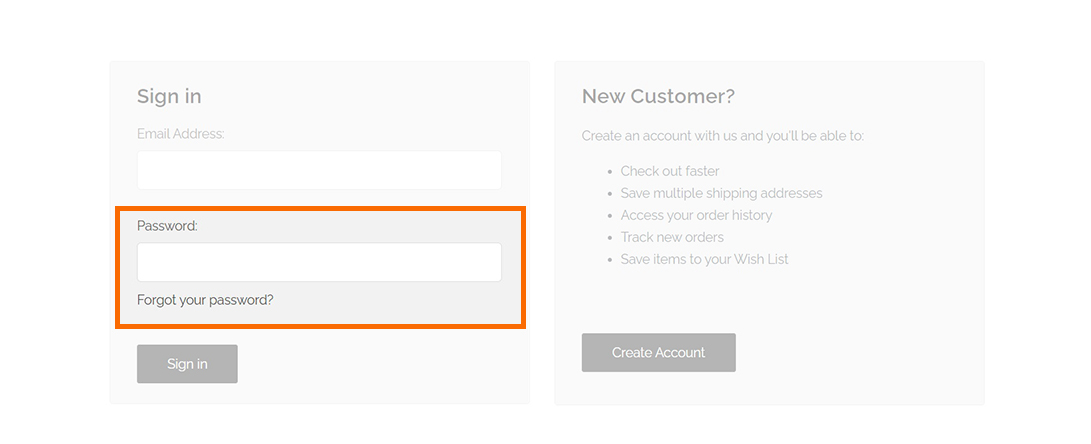The image is a screenshot of a typical login or sign-in page of a website, designed for users attempting to access their accounts for the first time. On the left side of the page, enclosed in a light gray box, is the sign-in section. The section starts with the heading "Sign-In" followed by the prompt "Email Address" with a corresponding white text input box below it. Beneath this, the prompt "Password" is displayed with another white text input box for the password entry. Below the password box, there is a link labeled "Forgot Your Password." The entire password section is highlighted with an orange-reddish outline, drawing attention to its importance. At the bottom of the sign-in section, there is a gray button labeled "Sign-In".

On the right side of the page, the focus shifts to new users with the heading "New Customer." It encourages new users to create an account, detailing the benefits such as faster checkout, saving multiple shipping addresses, accessing order history, tracking new orders, and saving items to a wish list. Below these benefits, a button labeled "Create Account" is prominently displayed, inviting users to register for the website.